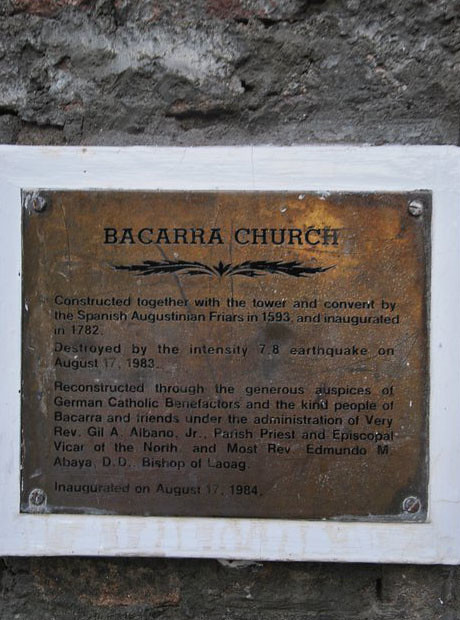The image is a tall, rectangular photograph of a dark gray stone wall with small bits of orange and white, taking up the top quarter and the bottom eighth of the image. Attached to the wall is a metal plaque bordered by a white wooden frame and fastened with four large screws, one at each corner. The plaque itself is copper-colored with black print. At the top, it reads "Baccara Church," followed by a feather-like separator. The inscription details the church's history: "Constructed together with the tower and convent by the Spanish Augustinian friars in 1593 and inaugurated in 1782. Destroyed by the intensity 7.8 earthquake on August 17, 1983. Reconstructed through the generous auspices of German Catholic benefactors and the kind people of Bacarra and friends under the administration of Very Reverend Gil A. Albano, Jr., Parish Priest and Episcopal Vicar of the North, and Most Reverend Edmundo M. Abaya, D.D., Bishop of Laoag. Inaugurated on August 17, 1984."